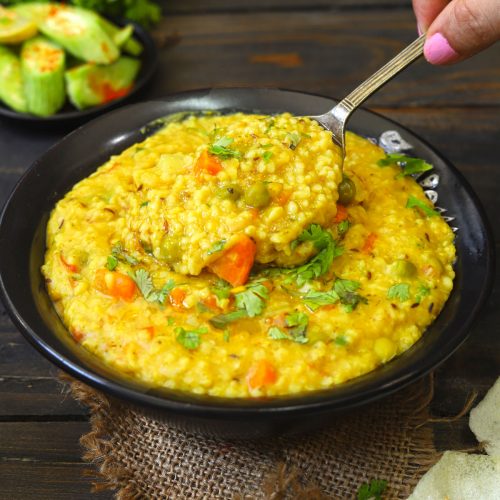This realistic square photograph captures a detailed scene on a rustic brown wooden plank table. At the center, a black bowl sits atop a piece of brown burlap or canvas cloth, filled with a thick, yellow soup, possibly corn chowder or a corn-based dish. The soup, rich with yellow hues, includes visible ingredients like sliced carrots and green vegetables, which could be cilantro or peas. A stainless steel spoon held by a person with pink fingernails dips into the bowl, capturing a spoonful of the hearty mixture. To the back left, a black plate showcases sliced fresh okra, softly blurred in the background. Toward the bottom right, a corner of a white cloth peeks into the frame, adding texture to this homely and appetizing composition.